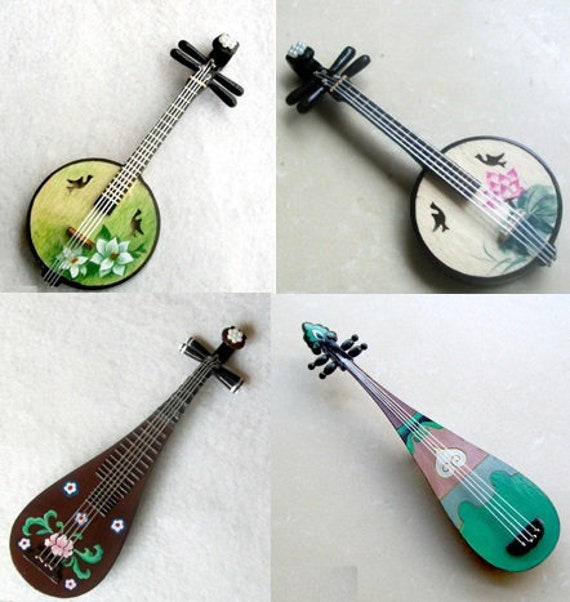The image is divided into four square pictures arranged in two rows and two columns, each featuring a unique musical instrument set against a light gray background. 

In the top left picture, a banjo with a predominantly green circular base adorned with a design of white flowers and green leaves, as well as two black birds, is shown. This banjo has white strings and a black handle with gold or white strips. 

The top right picture also features a banjo, characterized by a white circular base with a pink and white flower, green leaves, and two black birds. Its strings are white, and it has a black handle similar to the other banjo.

In the bottom left picture, there is a brown ukulele with an elongated body that is wider at the base. This ukulele has tan strings attached to a brown piece, and it is embellished with blue-outlined white flowers having red or brown centers, along with a pink flower with green leaves towards the bottom.

The bottom right picture showcases another ukulele with a colorful, elongated body. This ukulele features various shades like green, blue, pink, and purple. It also has white strings attached to a black piece, with the handle displaying a black section, a green and black strip, and a purple top.

Each instrument stands out against the light gray backdrop, highlighting their detailed designs and intricate patterns.